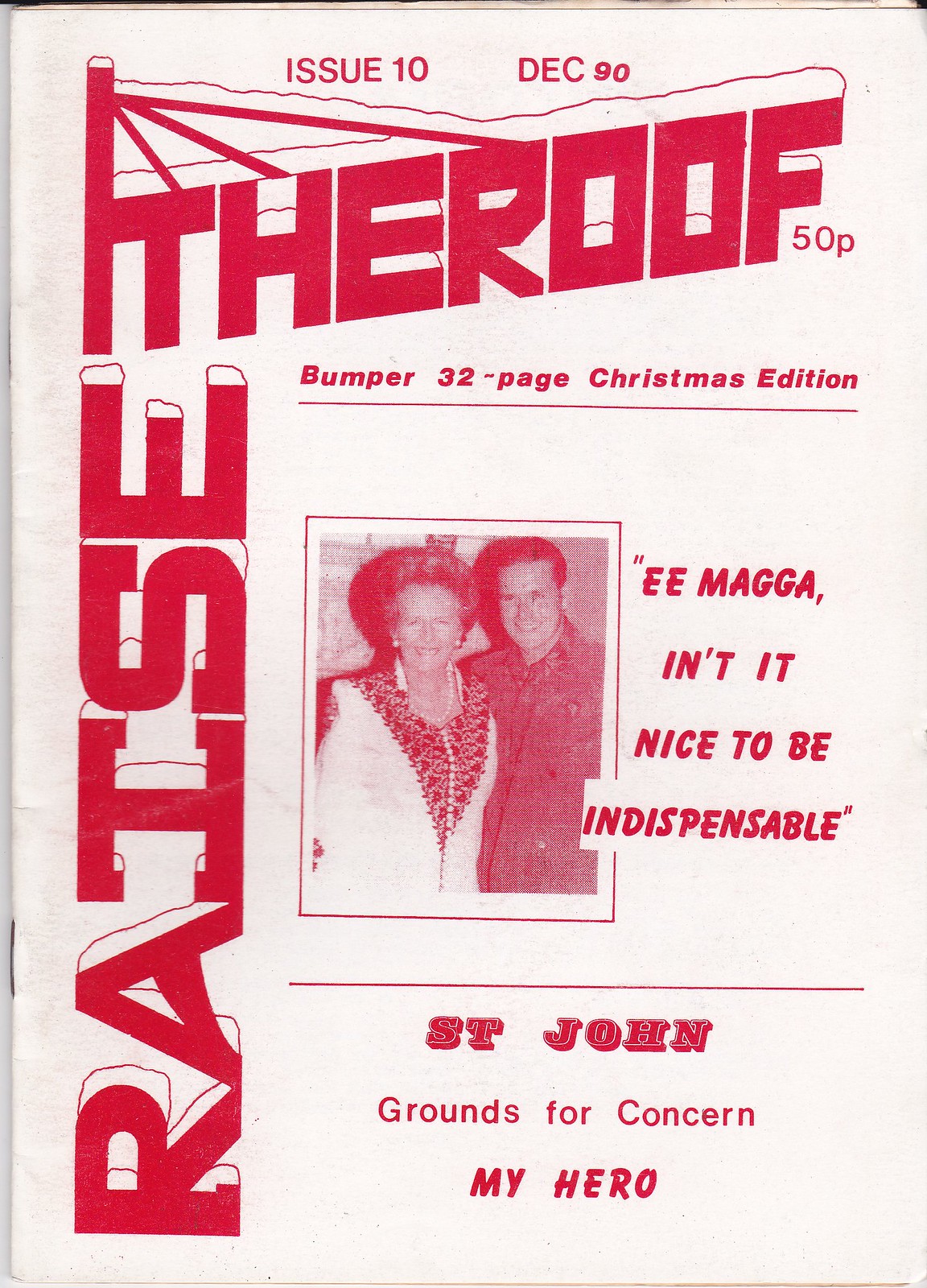This image is a detailed poster or program, possibly for a Christmas concert or play. It features a predominantly white background with prominent red lettering. At the very top, it reads "Issue 10, December 90" alongside "50p," indicating the price. The title "The Roof" is displayed in large red letters across the top, with “Raise” running vertically up the left side of the sheet, creating an inverse L-shape layout. A picture of a smiling man and woman appears in the center; the man is dressed in a dark shirt and the woman in a white dress. Adjacent to this image, there's a quote in red letters: "E.E. Maga, isn't it nice to be indispensable?" Below this quote, additional red text reads "St. John," followed by "grounds for concern" and "my hero," separated by a horizontal red line. This edition is highlighted as a "Bumper, 32-page Christmas edition." The entire composition suggests a festive theme and possibly a special Christmas issue, bound together by visible staples on the right edge.